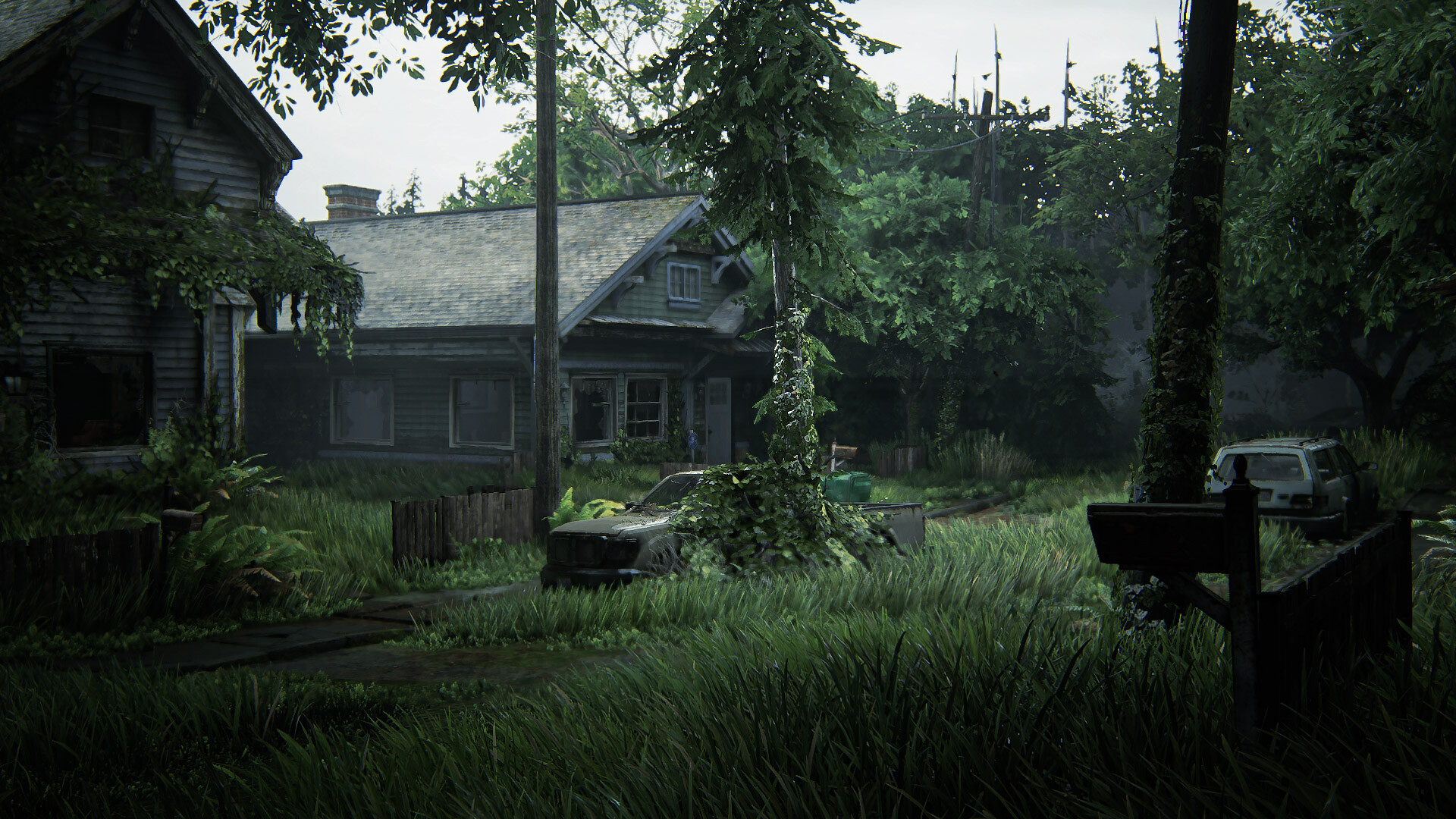The painting depicts a rural Southern setting characterized by two small, weathered houses flanking a narrow, overgrown sidewalk. The scene exudes neglect and abandonment, with tall grass and weeds encroaching on every corner. To the left, an old wooden building stands, shrouded in ivy and other vegetation, giving it a forlorn appearance. Its dilapidated state is matched by the dated look of a nearby second house that, while also rundown, appears to have seen more recent habitation, evidenced by its trimmed lawn. The windows of this second house tell a story of time and hardship; some are boarded up while others remain glass-fronted. Between the taller house and the shorter one, an old truck and another car can be seen, seemingly abandoned, adding to the desolate atmosphere. The scene is framed by assorted tall trees and the sky above is grey, heightening the sense of neglect pervasive throughout this deserted neighborhood.